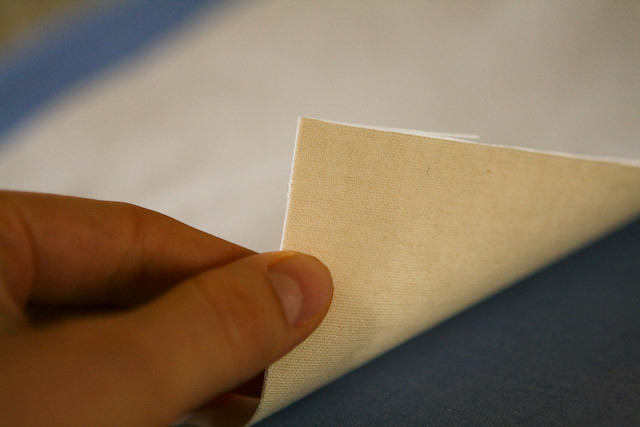This detailed photograph captures a close-up of a person's left hand lifting a piece of beige, tweed-like fabric, revealing its underside. The hand, visible from the lower quarter of the image, uses the thumb and forefinger to hold the fabric, which is tilted upward from a table. The texture of the fabric appears slightly rough and durable, and the neutral color suggests it could be used as a tablecloth, upholstery material, or another type of covering. The background is out of focus, emphasizing the hand and fabric, while the table surface underneath can be faintly seen. The scene slightly resembles the motion of turning a page, with the fabric forming a triangle opposite the hand and the background appearing to have a dark blue hue.